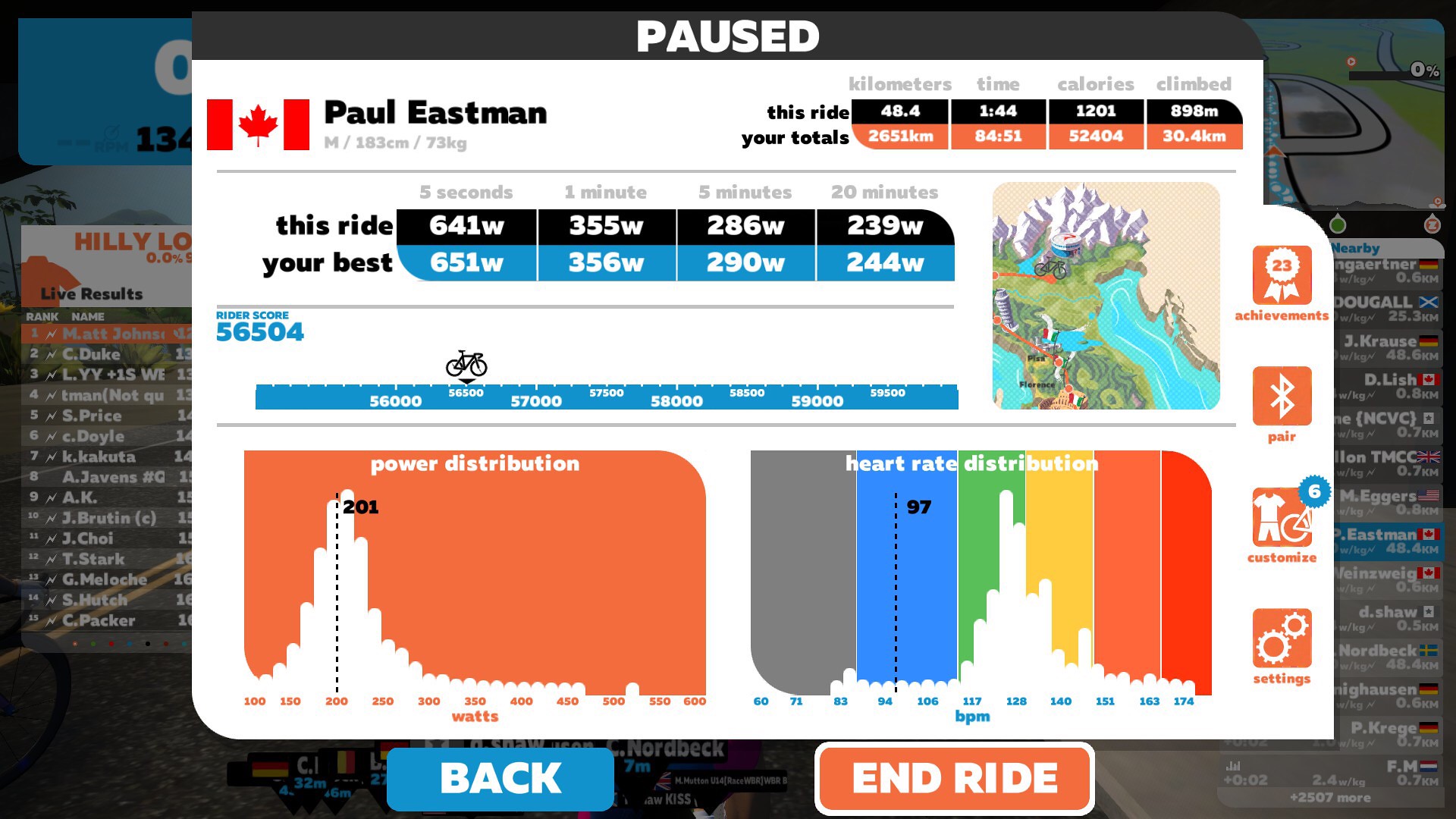This image shows a paused screen from an electronic exercise device, likely a Peloton bike. At the top center, "Paused" is displayed in white letters on a gray background. The main focus is a detailed overlay that presents performance stats for a user named Paul Eastman from Canada, indicated by a Canadian flag. 

On the left, "Hilly" is listed alongside live results and various names, indicating competitors or previous rides. On the right, "Nearby" shows names with associated flags. The overlay highlights multiple performance metrics: "This Ride" and "Your Totals" in black and coral-colored blocks respectively. 

Key stats include:
- **This Ride:**
  - Distance: 48.4 km
  - Duration: 1 minute 44 seconds
  - Calories: 1,201
  - Elevation: 898 meters

- **Your Totals:**
  - Distance: 2,651 km
  - Duration: 84 minutes 51 seconds
  - Calories: 52,404
  - Elevation: 30.4 km

Power output is detailed in black and blue boxes with white fonts, comparing "This Ride" to "Your Best" over various durations:
- **This Ride:** 641W (5s), 355W (1 min), 286W (5 min), 239W (20 min)
- **Your Best:** 651W (5s), 356W (1 min), 290W (5 min), 244W (20 min)

To the right is a topographical map showing the route. Below, in coral and blue boxes, there are metrics for power distribution highlighting 201 and heart rate distribution with 97 in gray, blue, green, yellow, coral, and orange.

At the bottom left, a blue button labeled "Back" and on the right, an orange button labeled "End Ride" are displayed. Additional details include rider score progress of 56,500, achievements (23), Bluetooth connectivity, customization (6), and access to settings. The screen effectively tracks and displays detailed ride statistics and performances.